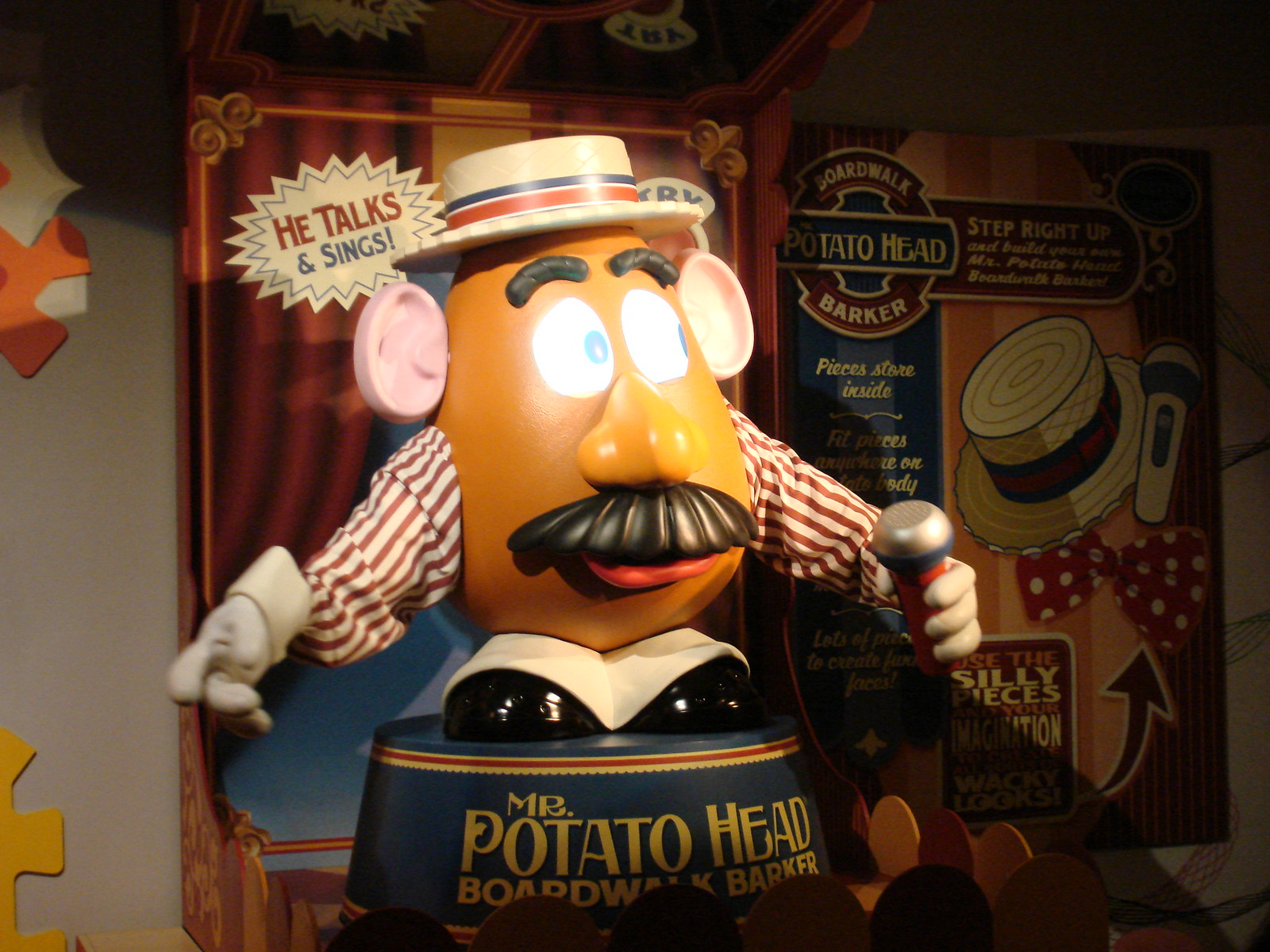The photograph showcases an intriguingly detailed toy, a whimsical interpretation of Mr. Potato Head designed as a Boardwalk Barker. This plastic Mr. Potato Head features a stylized human face with large white eyes, blue pupils, and black curved eyebrows beneath an old-fashioned barbershop straw hat adorned with a red, white, and blue band. Adding character are his oversized pink ears and a distinctive black mustache above pink lips. 

Instead of a traditional potato body, this toy has robotic-looking arms and shoes covered in white cloth, reminiscent of a circus performer’s getup. He stands on a small platform labeled "Mr. Potato Head Boardwalk Barker," illuminated by a spotlight accentuating the details. Behind him, cardboard packaging promotes his interactive features with phrases like "He sings and talks" and "Try me" accompanied by a large red button. The overall design, including long arms bearing a stripe pattern akin to barbershop quartet attire, conveys a vintage circus aesthetic, complete with the suggestion to "use the silly pieces and your imagination to make wacky looks." This playful yet intricate rendition captures the essence of a singing, talking Mr. Potato Head, styled as a charismatic carnival barker ready to entertain.